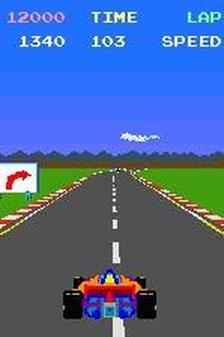This screenshot is from the classic video game "Pole Position," known for its retro graphics and formula racing gameplay. In the image, a vividly colored racing car—featuring shades of orange, blue, and red—resembling a Formula 1 vehicle, is positioned at the center of the gray asphalt track. The edges of the track are adorned with a distinctive white and red pattern. On the left side of the screen, an indicator signals an upcoming turn in the track. The background is a picturesque blue sky coupled with a distant line of trees lining the horizon. At the top of the screen, various game metrics are displayed, including the player's score, time, current lap, and speed, providing an authentic vintage gaming experience.